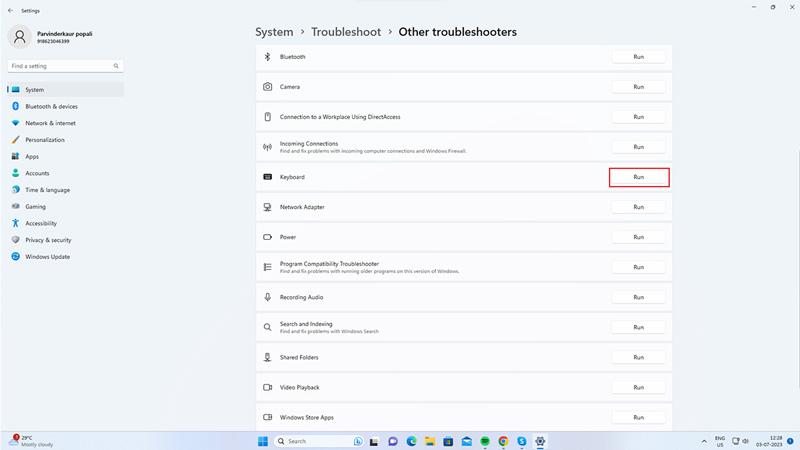The image depicts a Windows settings page focused on troubleshooting options. At the top, the title reads "System" followed by subheadings "Troubleshoot" and "Other Troubleshooters." Below this, there is a long list of troubleshooting items, each housed in a white box. These items are:

1. **Bluetooth**
2. **Camera**
3. **Connection to a Workplace using Direct Access**
4. **Incoming Connections**
5. **Keyboard** (notably highlighted with a red box next to it)
6. **Network Adapter**
7. **Power**
8. **Program Compatibility Troubleshooter**
9. **Recording Audio**
10. **Search and Indexing**
11. **Shared Folders**
12. **Video Playback**
13. **Windows Store Apps**

Each item has a "Run" button on the right-hand side, allowing users to initiate troubleshooting.

At the top left, there is an unpronounceable name, accompanied by a search box labeled "Find a setting." On the left side of the page, there is a vertical list of different tabs labeled:

- System
- Bluetooth and Devices
- Network and Internet
- Personalization
- Apps
- Accounts
- Time and Language
- Gaming
- Accessibility
- Privacy and Security
- Windows Update

This detailed breakdown provides a comprehensive view of the various troubleshooting options available in this Windows settings section.